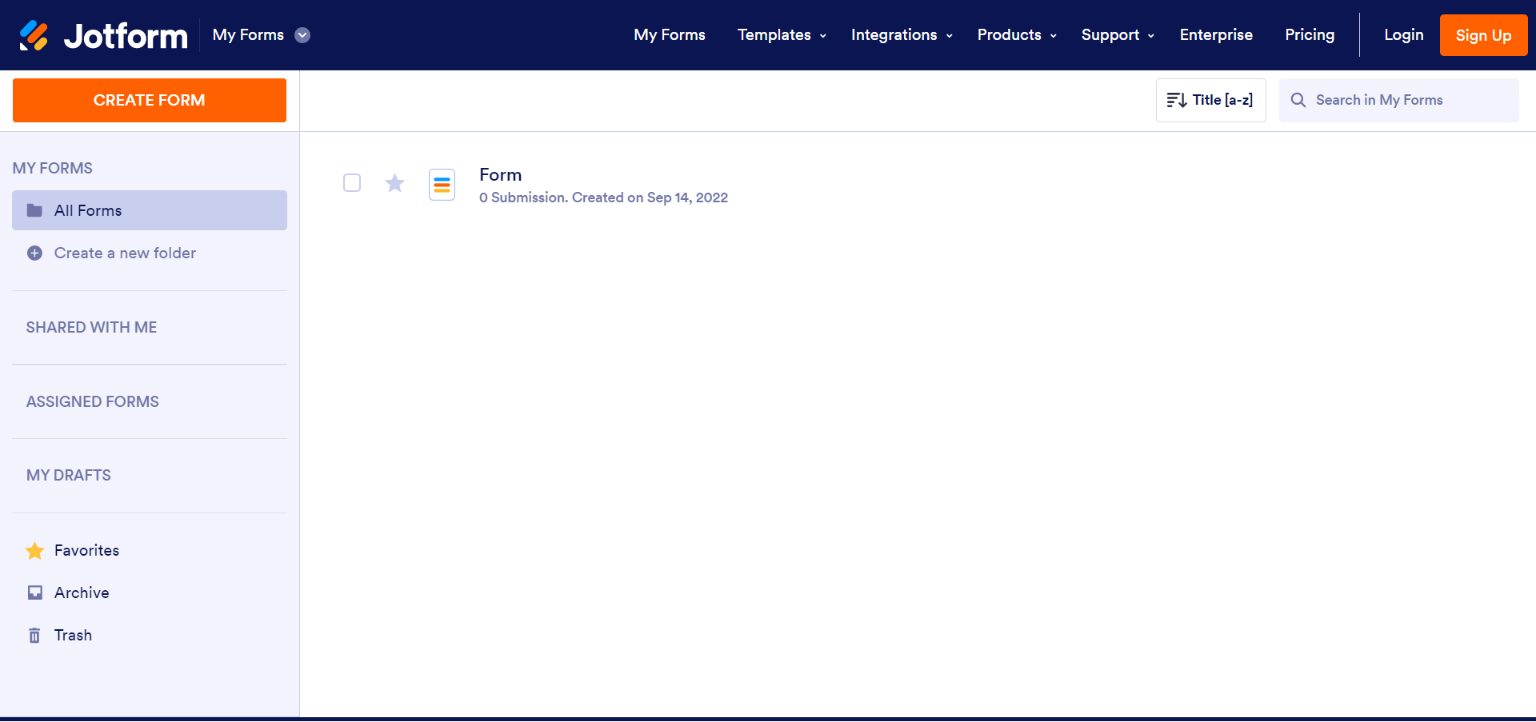The image depicts a section of a web page with a primary focus on the layout and navigation options of a form-building platform, JotForm. At the top of the page, there is a dark blue navigation bar. In white text, the bar displays "JotForm," followed by a circle with a checkmark labeled "My Forms," and links to "Templates," "Integrations," "Products," "Support," "Enterprise," "Pricing," and "Login." Next to these, an orange rectangle with white text reads "Sign Up."

On the main part of the page, to the left, an orange rectangle contains the text "Create Form." To its right, there are sorting options "Title A to Z" and a search function labeled "Search in My Forms."

To the far left, a vertical blue rectangle lists several navigation options in white text: "My Forms," "All Forms," "Create a New Folder," "Shared with Me," "Assign Forms," "My Drafts," "Favorites," "Archive," and "Trash."

On the right side of the page, there is a list of individual forms. Each entry shows the form name, the text "Zero Submissions," and the creation date "September 14, 2022." A small icon depicting a piece of paper with colorful lines accompanies each form entry.